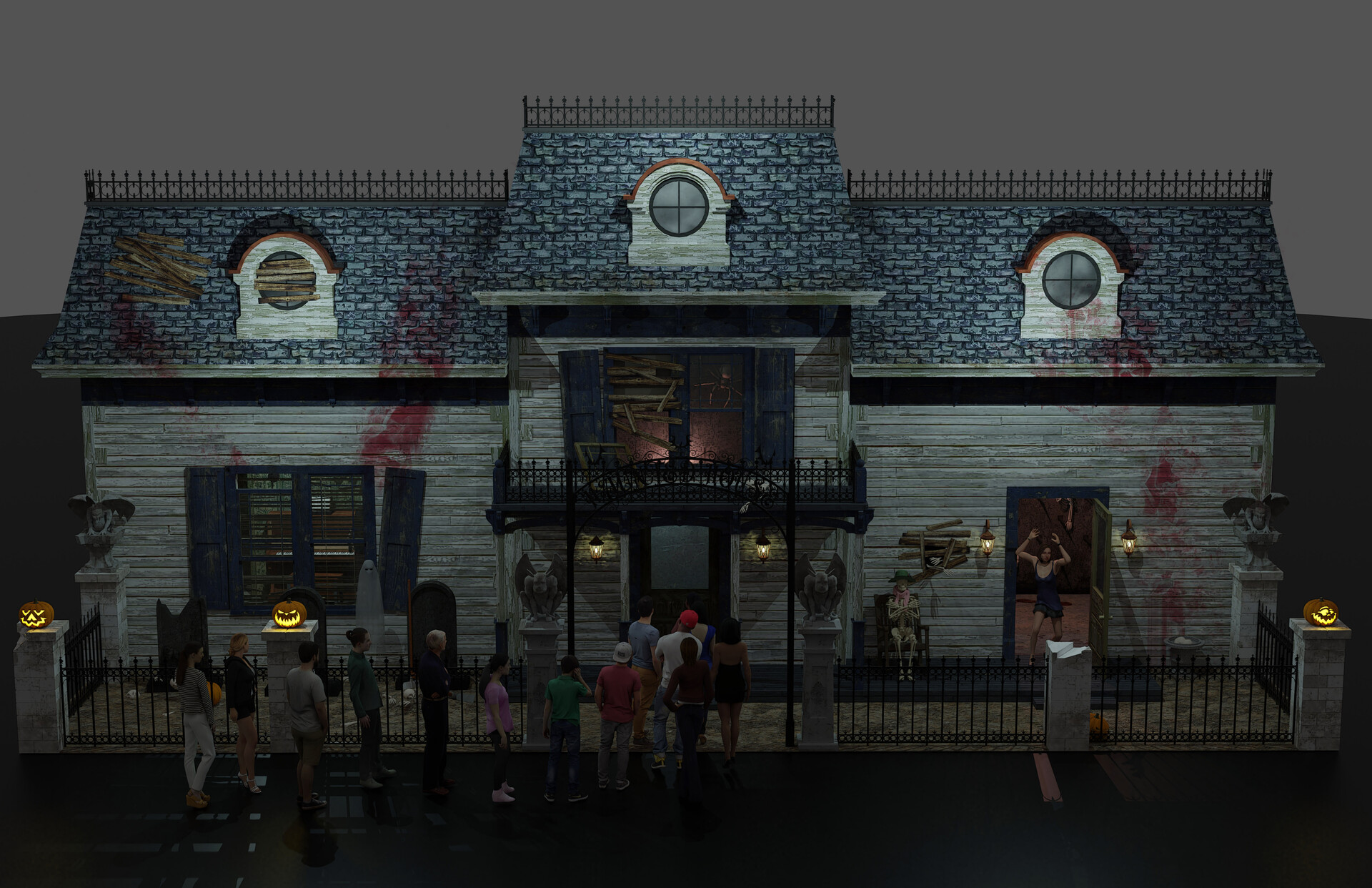This computer-generated graphic showcases a spooky haunted house set against a grayish, ominous background. The decrepit structure features boarded-up windows and eerie bloodstains across its wooden or white side paneling. The blue-tiled roof is adorned with anti-pigeon spikes, and a balcony on the second story emits a faint light from a room with boarded windows and a giant spider in the middle window.

At the front of the house, a line of diverse individuals, including women in scanty dresses, men in casual attire, and an elderly person, anxiously wait their turn to enter. Two gargoyles guard the entrance, flanked by an iron fence. Detailed decorations enhance the creepy atmosphere: jack-o'-lanterns with various expressions sit atop white pillars, although one pillar is entirely broken. An unsettling scene unfolds to the right of the door, where a skeleton in a green hat and pink scarf sits on a chair. Nearby, a woman with her hands up, possibly dancing or frightened, stands next to a wall displaying a severed arm and additional blood splatters.

The entire setup, resembling a Halloween game environment, presents a chilling but fascinating ambiance, complete with meticulously crafted elements that make the haunted house disturbingly lifelike.